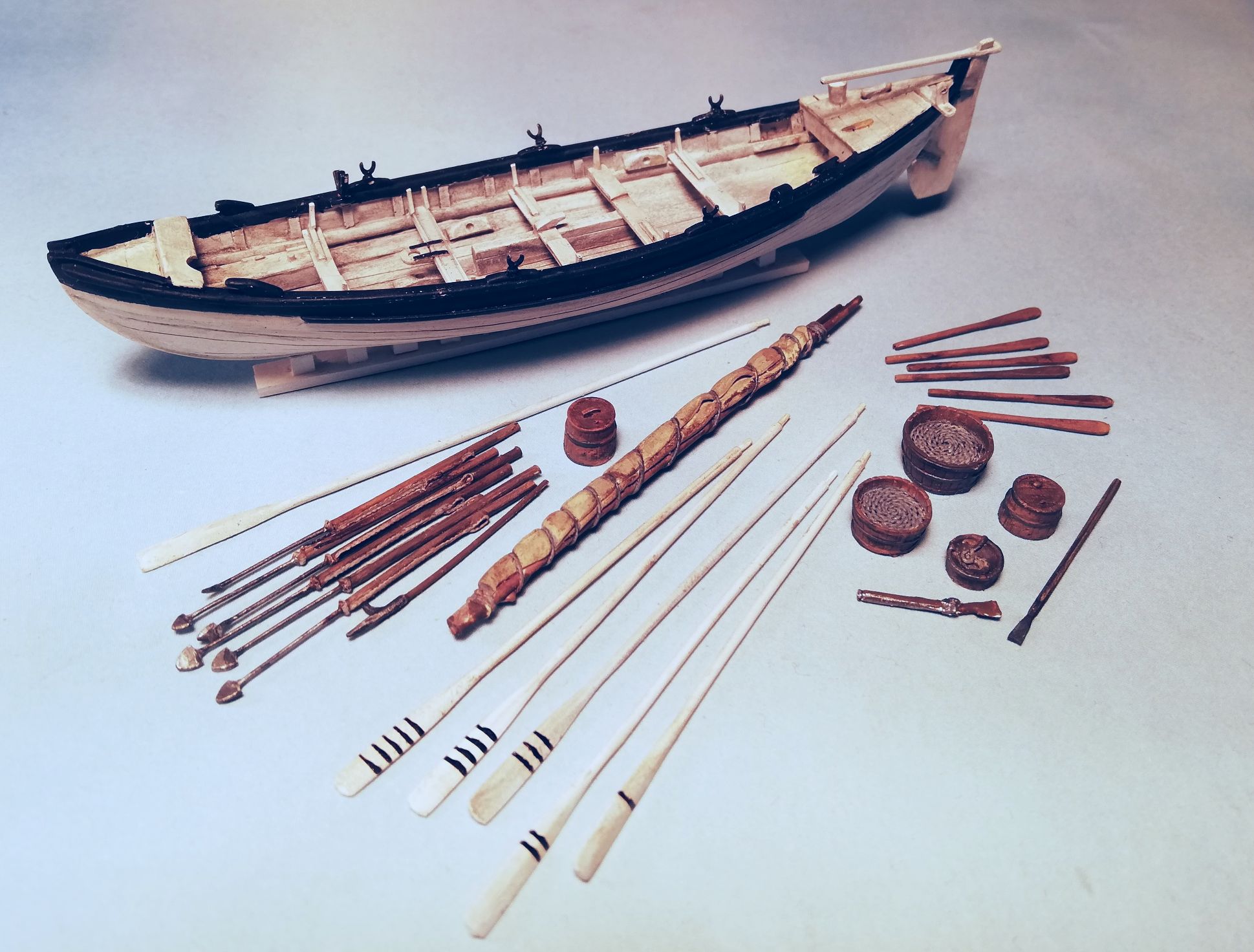The image showcases an unassembled wooden boat model kit set against a gray background. The kit prominently features a partially completed boat in the background, characterized by a brown wooden body and a black border around the top edge. Scattered in front of the boat are numerous small parts necessary for assembly, including various wooden rods, dowels, and toothpick-like pieces. These parts range in color, primarily in shades of brown, with a few white sticks interspersed. Notably, there are several paddles marked with black stripes, extending from one to five marks, lying near the front and sides. Additionally, the kit includes small round pieces, several metal tools, and miniature wooden buckets, all arranged meticulously around the primary components, emphasizing the intricate detail and comprehensive nature of the model-building process.